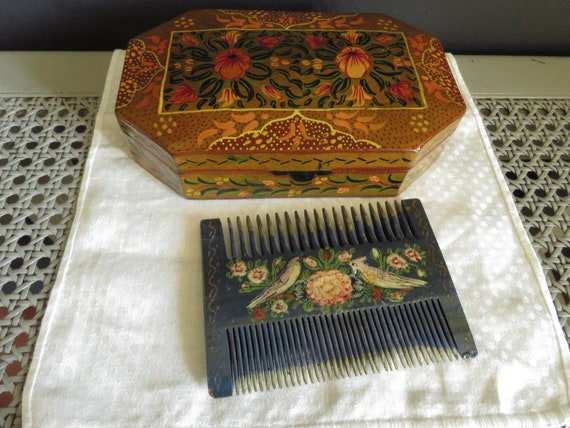The image showcases a beautifully ornate and elaborately decorated wooden box, characterized by intricate floral patterns in hues of pink, yellow, red, and green, set against a brown, mustardy background. Beside the box rests an antique-looking blue comb, adorned with paintings of two birds amidst a central large flower and several smaller flowers in pink, white, and green. The comb has tooth variations: fine teeth on one side and wider, coarser teeth on the other, intended for different stages of hair grooming, which suggests it was a prized possession. This setup, which hints at a gift given to a girl or young woman from a wealthy background, perhaps in the 1700s or 1800s, is placed on a white, wicker-like woven surface with a white cloth featuring circular patterns. The attention to detail in both the box and the comb highlights their antique and possibly expensive nature, making them likely cherished items from their era.